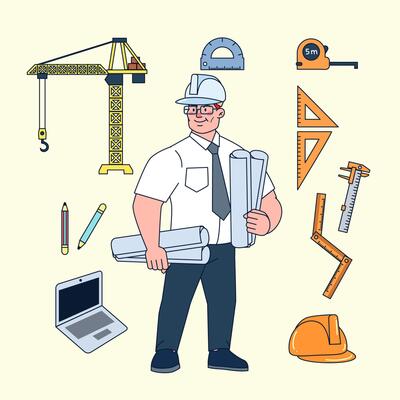This cartoon-style illustration portrays an architect or engineer at the center of the image, dressed in a white button-up shirt with a gray tie and blue pants, wearing a hard hat. He is smiling and holding several reams of blueprints under his arms. Surrounding him are various work-related items that reinforce the engineering theme, including a laptop, pencils, pens, rulers, a protractor, a ruler’s compass, and two triangles. A yellow crane and an orange hard hat are also visible in the background, alongside a tape measure marked with "5m." The overall scene is set against a yellow background, creating a vibrant and professional atmosphere. This detailed illustration would be well-suited for use in engineering blogs, articles, or corporate materials related to construction and design professions.